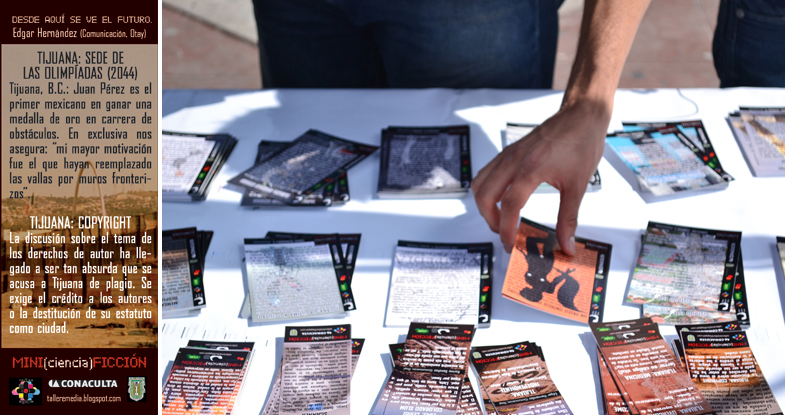The photograph captures a white table set up outdoors, bathed in sunlight and casting the shadows of onlookers in the foreground. On the table, a collection of cards and pamphlets is spread out, displaying various illustrations and texts primarily in Spanish. Dominating the left side of the frame is a brown vertical bar featuring the headline "Tijuana, Sede de las Olimpiadas 2044," followed by text about Juan Perez, the first Mexican to win a gold medal in a hurdling event. The cards and pamphlets appear to be advertisements or promotional materials related to a science fiction narrative involving Juan Perez in a futuristic Tijuana. In the center, a right hand reaches down to pick up one of these cards, further highlighting the interactive nature of the display. The overall scene suggests a dynamic public engagement, possibly at a community event or a promotional gathering.